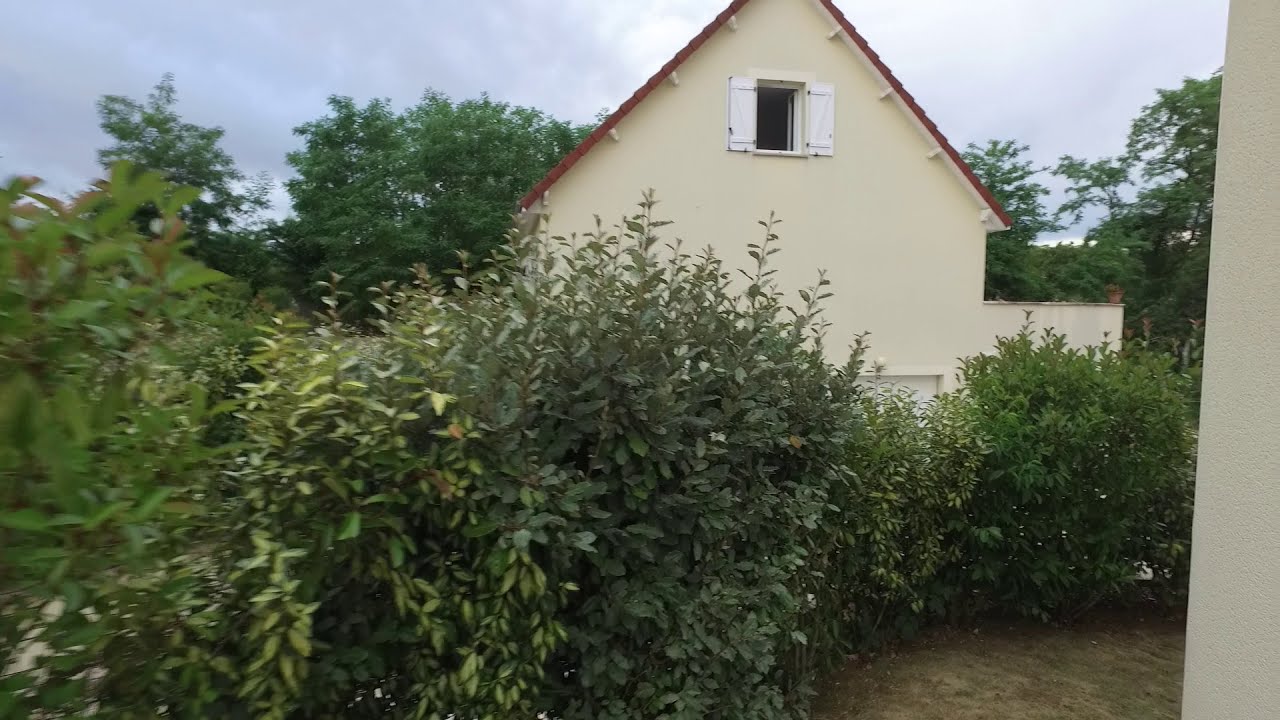The image captures a residential setting, with a focus on the side of a two-story house positioned towards the right side of the frame. The house features a tan cream-colored exterior with an A-shaped roof adorned with red tiles. There is a single, upper-story window, likely in the attic area, flanked by white shutters, which offers a stark contrast to its dark interior. Bushes form a dense wall in the foreground, partially obstructing the lower part of the house, which might include features like a garage, though these are not clearly visible. A small section of grass is noticeable in the bottom right corner, adding a touch of greenery. Behind the house, additional trees are visible, complemented by a cloudy sky that occupies the top edge of the image. The camera angle, set approximately six feet high, suggests the picture was taken from outside another house, with a partial view of a wall or pillar on the right side, indicating a neighborly proximity.